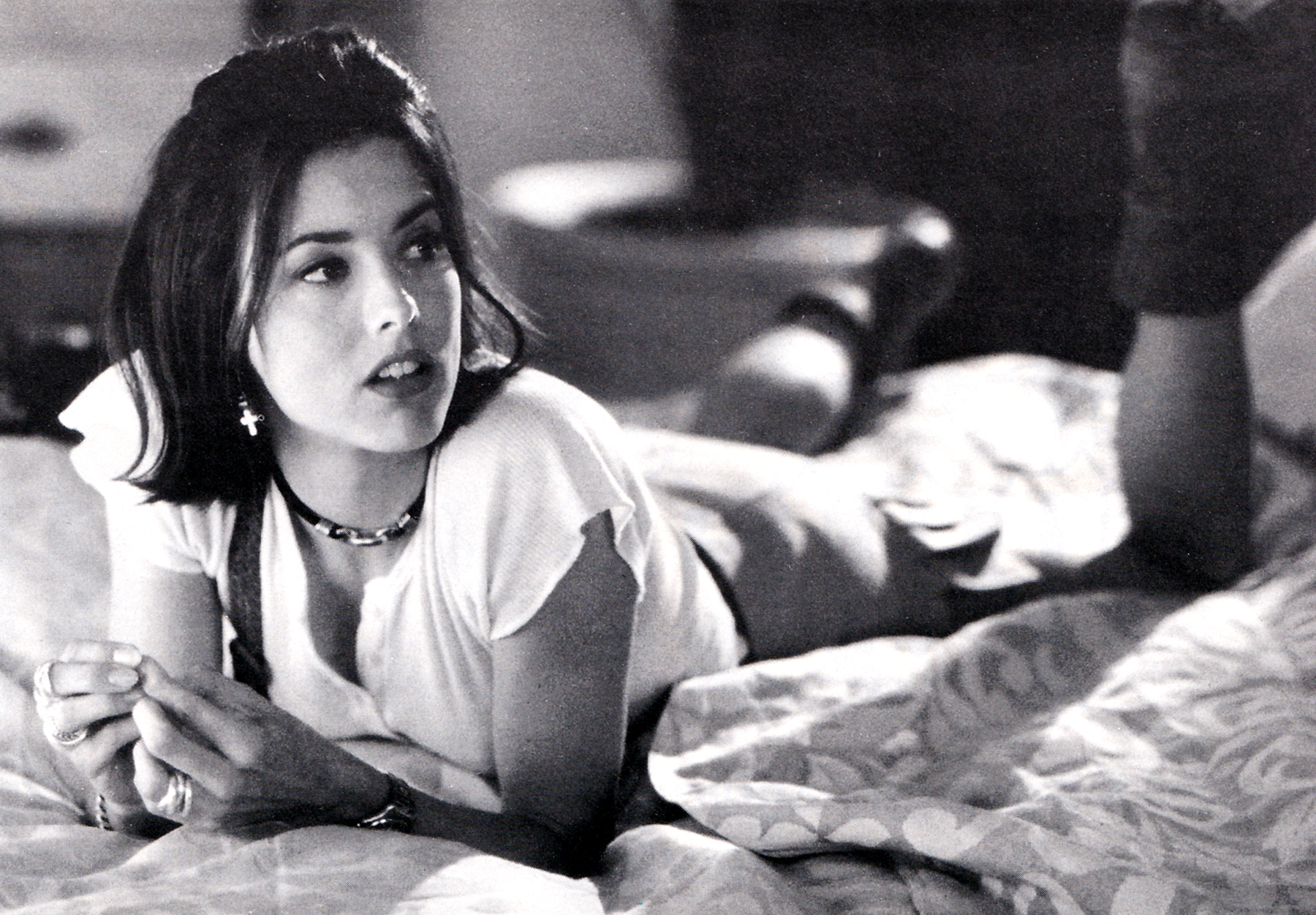The black and white image captures an indoor scene, likely set in a bedroom. Dominating the composition, a bed extends horizontally across the center of the frame. A woman with black hair is lying on her stomach on the bed, turned slightly to the right side of the image. Her attire includes a white shirt paired with a skirt, and she is wearing calf-high boots. Accessories such as cross earrings, a necklace, and either a bracelet or a watch are also visible. The background appears blurred, revealing indistinct furniture and potentially a flower pot, which is out of focus.